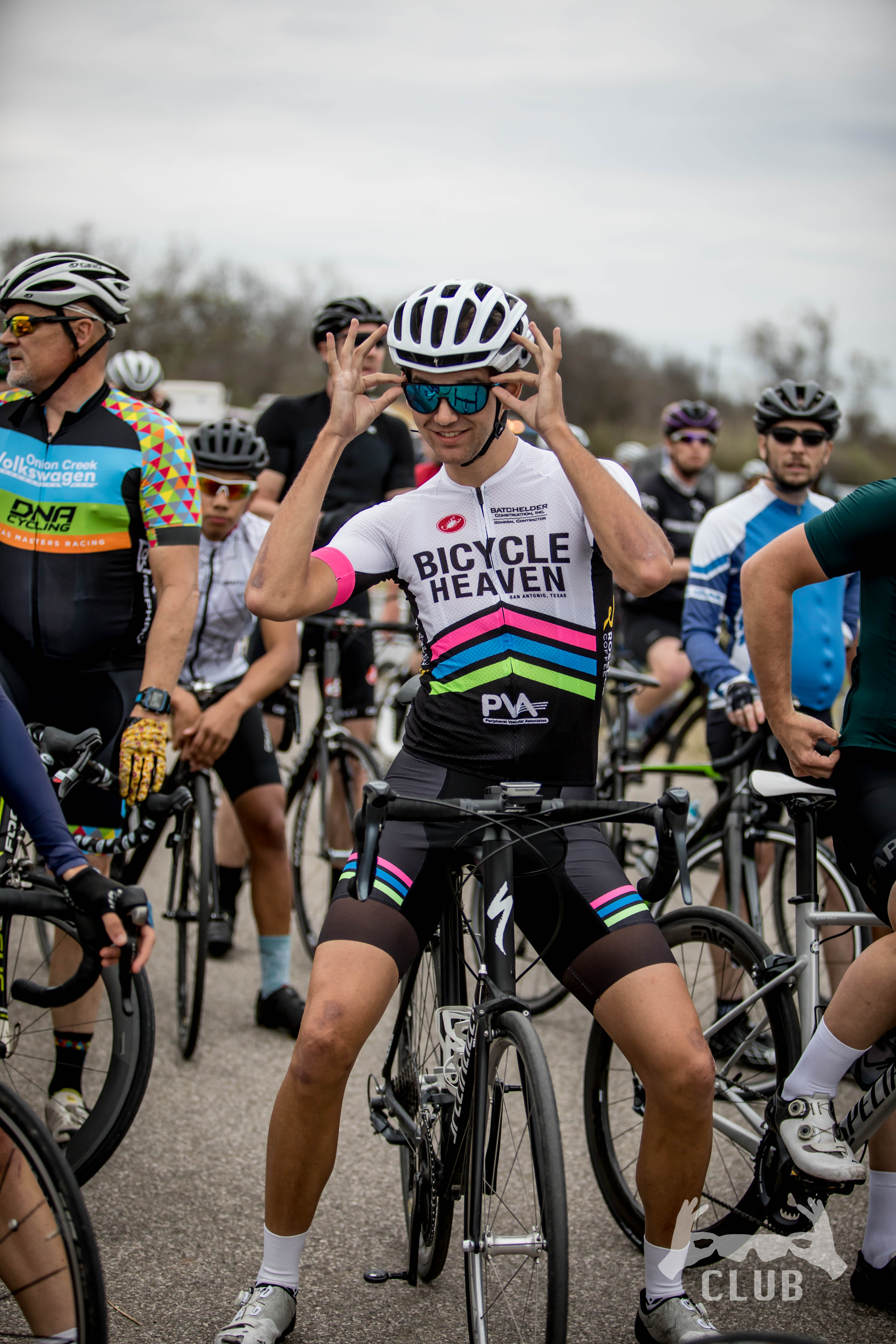In the photograph capturing the beginning of a bike race, a crowd of male cyclists are gathered together, either seated or standing beside their bicycles, waiting for the event to start. They are all dressed in racing gear, complete with biking shorts, shirts, and helmets featuring multiple air vents. Dominating the center of the image is a cyclist with sunglasses and a distinctive white helmet adorned with three neon stripes—pink, blue, and neon green. His jersey, which reads "Bicycle Heaven," mirrors this color scheme and extends onto his shorts. To his left stands an older man, also wearing a ventilated helmet, dark sunglasses, and a predominantly black jersey with polka dots on the shoulders and sleeves. Amidst these cyclists, one man leans disinterestedly on his handlebars, waiting for the race to commence. In the background, more cyclists and a slightly overcast sky framed by distant trees are visible. A logo featuring a pair of sunglasses and the word “club” is displayed at the bottom right, reflecting the pose of the central cyclist adjusting his own sunglasses.